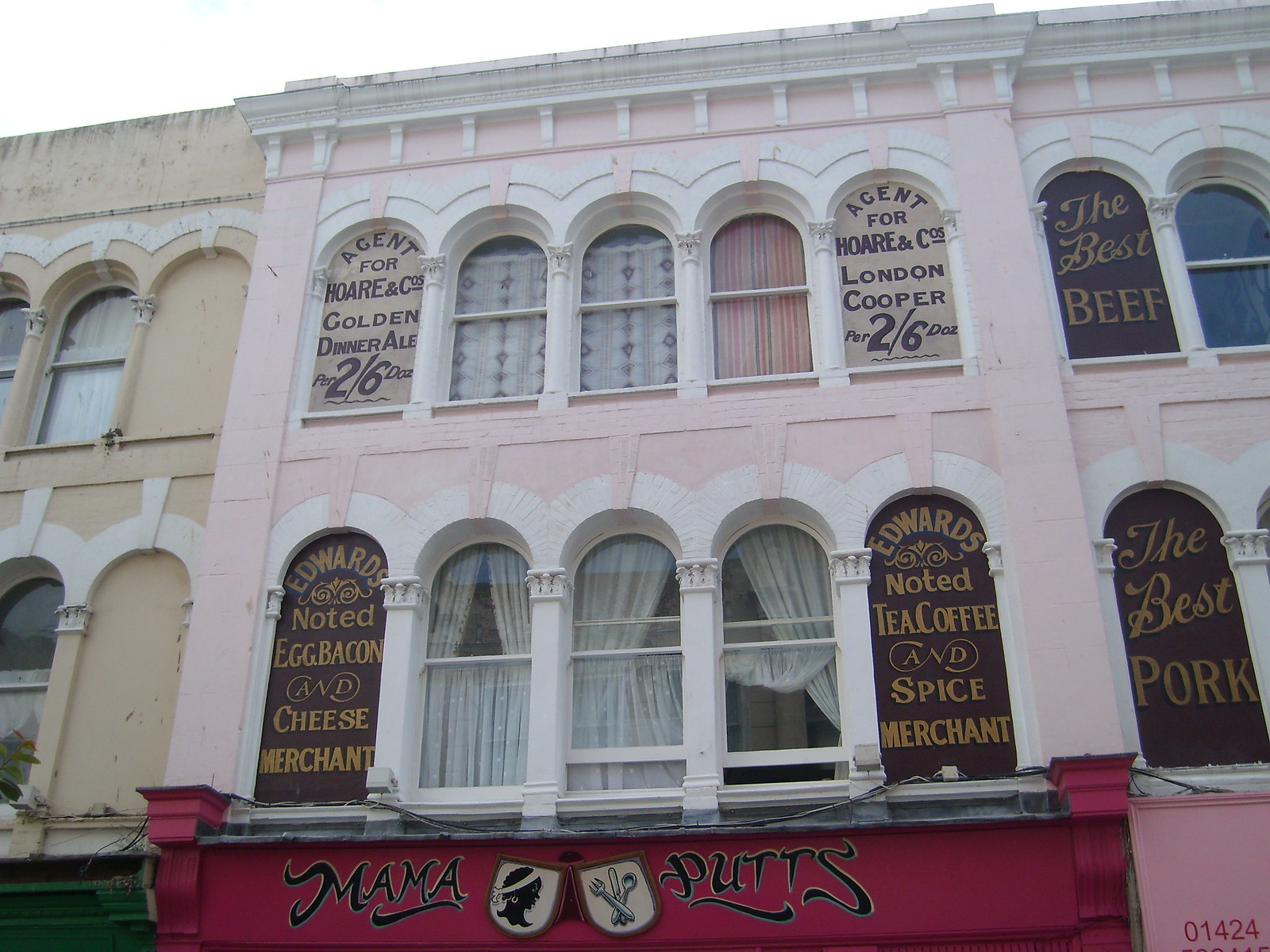This image depicts the side of a tall, rectangular building with a mix of architectural and commercial elements, viewed from a slightly upward angle. At the bottom center of the image, a vibrant red banner reads "MAMA PUTZ" in bold black letters, flanked by two symbols: a fork, knife, and spoon, and the profile of a woman with a white headband.

The building itself is comprised of two stories, each with five arched windows. The central portion showcases three windows with white curtains, while the left and right windows on both stories display various brown and tan signs. These signs advertise several offerings, including “Edwards Noted Egg, Bacon, and Cheese Merchant,” “Agent for Hoar and Co.'s Golden Dinner Ale per two/6 DOZ,” “The Best Beef,” “The Best Pork,” and “Edwards Noted Tea, Coffee, and Spice Merchant.”

The first building appears brown with white window framing and is seamlessly attached to a second pink and white building, featuring similar window styling. The sky is visible at the very top of the image, adding a bright, white backdrop. Each window's framing and signage contribute to the intricate architectural design typical of city buildings, emphasizing the commercial presence in this urban setting.